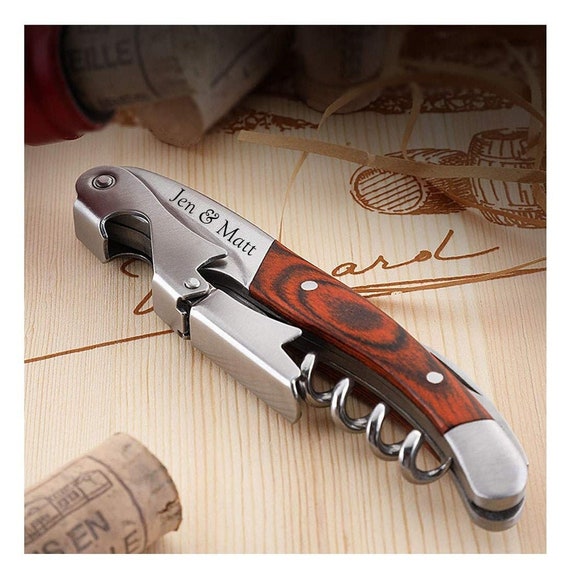This image features a close-up of a vintage, custom-made knife with a wood grain handle, elegantly engraved with "Jen & Matt" in black lettering. The knife is multifunctional, equipped not only with a blade but also with an integrated corkscrew for opening wine bottles and a potential bottle opener feature. The knife rests on a wooden table adorned with illustrations of wine barrels, and nearby, a cork can be seen. The craftsmanship includes several rivets and the wooden handle showcases varied grain patterns. This detailed image highlights the functional and aesthetic qualities of the knife, making it a memorable gift, likely intended for Jen and Matt.